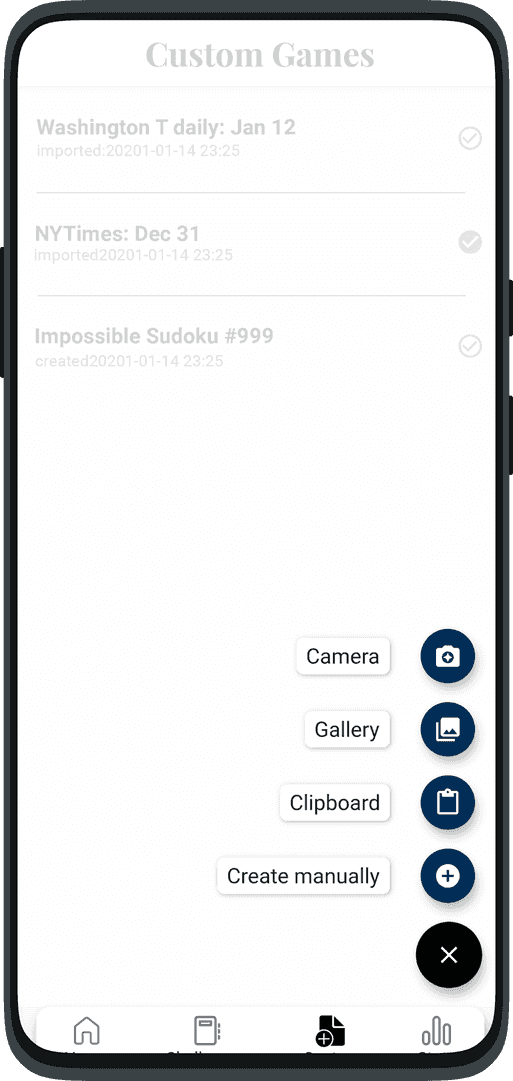In this image set against a white background, we see a black cell phone with the screen on. The phone has two buttons on its right side; the top button is smaller and shorter than the one beneath it. On the left side, there is one long black button. The screen displays a footer at the bottom with icons arranged from left to right in gray: a home icon, a gas tank, a page, and three vertical lines. At the top of the screen, light gray text reads "custom games." Below that, it says "Washington T. Daily January 12th" with a small circle containing a check mark to the right. Further down, it states "Imported 2021 114 23 25." Below this, there is another text entry that reads "New York Times December 31st," with the check mark now in a black circle.